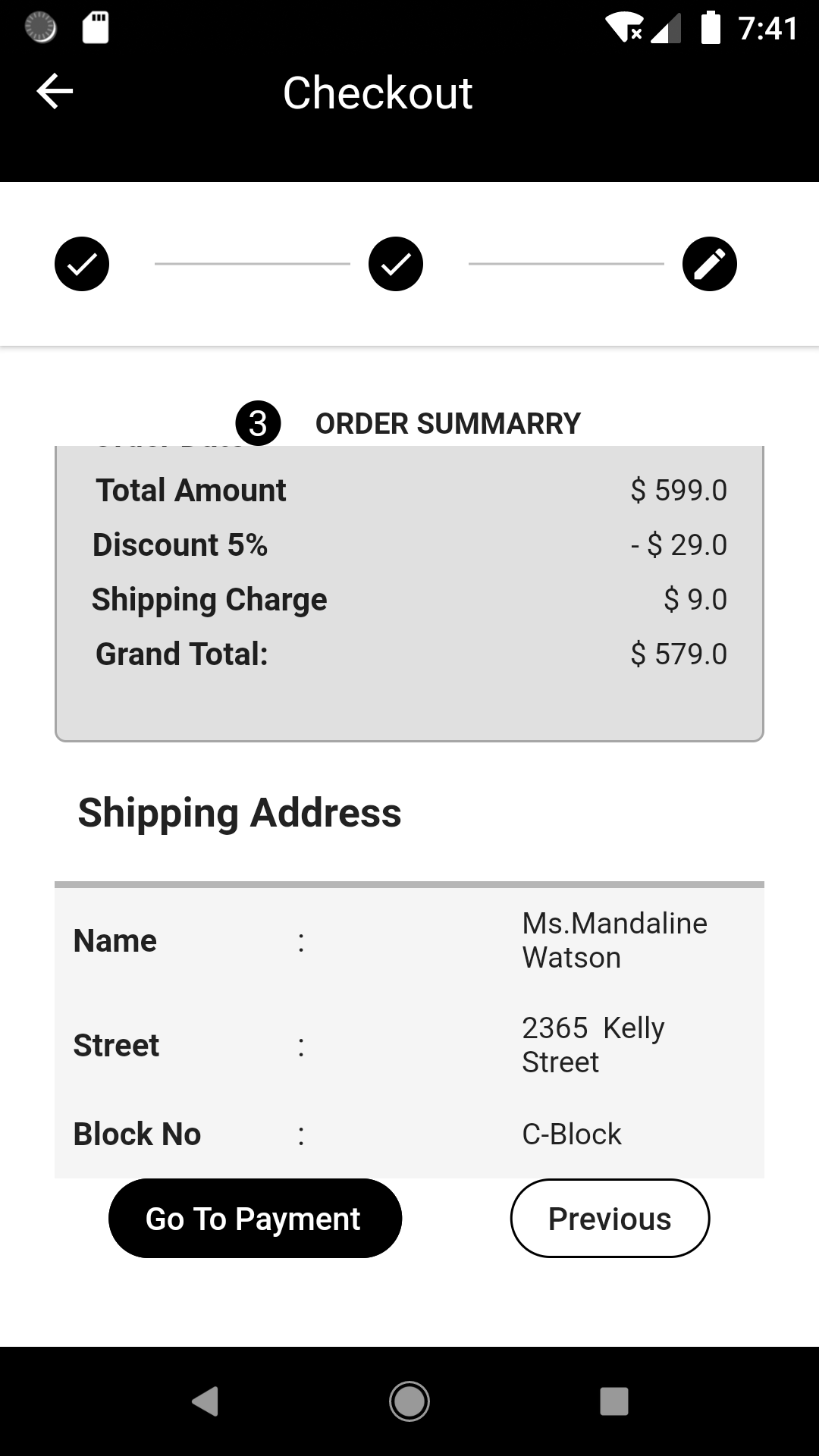This is a detailed screenshot of a mobile phone screen displaying a checkout page within an app. 

At the top left, a back arrow is visible on a black header bar, followed by the word "Checkout" centered in white text. The header bar also contains white icons on the right, including a Wi-Fi signal icon with an X over it, indicating no Wi-Fi connection, a half-filled phone signal icon, a full battery icon, and the time, which reads 7:41.

Directly beneath the header, there are three evenly spaced black circles. The two circles on the left contain white check marks, indicating completed steps. The third circle on the right has a pencil icon, denoting the current step. Below these circles, a larger black circle with the number "3" signifies the current step, labeled "Order Summary."

The main content of the page includes a gray rectangle that itemizes the order details: the total amount is $599, a 5% discount reduces this by $29, and a shipping charge of $9 is added, leading to a grand total of $579.

Following this, the shipping address is displayed in another gray rectangle, detailing the recipient’s name as Miss Madeline Watson, the street address as 2365 Kelly Street, and the block as C Block.

At the bottom of the screen, there are two prominent buttons for navigation. On the left, a black button labeled "Go to Payment" in white font, and on the right, a white button labeled "Previous" in black font.

Finally, at the very bottom of the screen, you can see the standard navigation icons for the device: a back button, a home button, and a square icon whose function is unclear from the description provided.